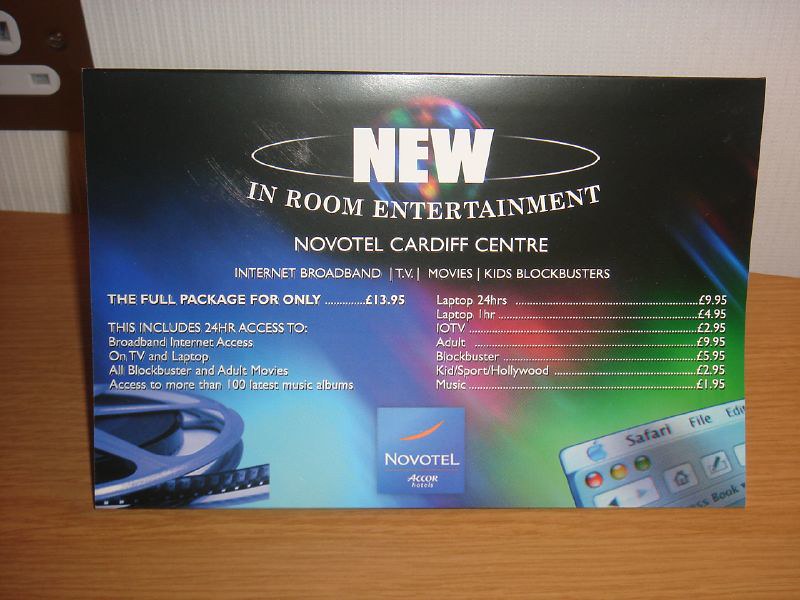The image captures an advertising card for in-room entertainment at the Novotel Cardiff Center, likely taken inside a hotel room. The card, set on a wooden table against a white wall with a switchboard, promotes a comprehensive entertainment package. At the top, in large white capital letters on a black background, is the word "New," followed by "In-Room Entertainment" in smaller font and the hotel name, "Novotel Cardiff Center." The card is colorful, with shades of blue, pink, red, and green, and features a picture of a film reel. The bottom center displays the Novotel Aircore logo in a blue square box, and there is an image of a computer screen with Safari browser icons.

The entertainment package is priced at £13.95, offering 24-hour access to high-speed broadband internet on TV and laptop, all blockbuster and adult movies, and more than 100 of the latest music albums. Specific pricing details include: 
- £9.95 for 24-hour laptop access
- £4.95 for 1-hour laptop access
- £2.95 for IOTV
- £9.95 for adult content
- £5.95 for blockbuster movies
- £2.95 for Kids Blockbusters
- £1.95 for music access

This detailed breakdown is presented with various price points on the right and left sides of the card, making it clear that the package caters to a wide range of entertainment needs.